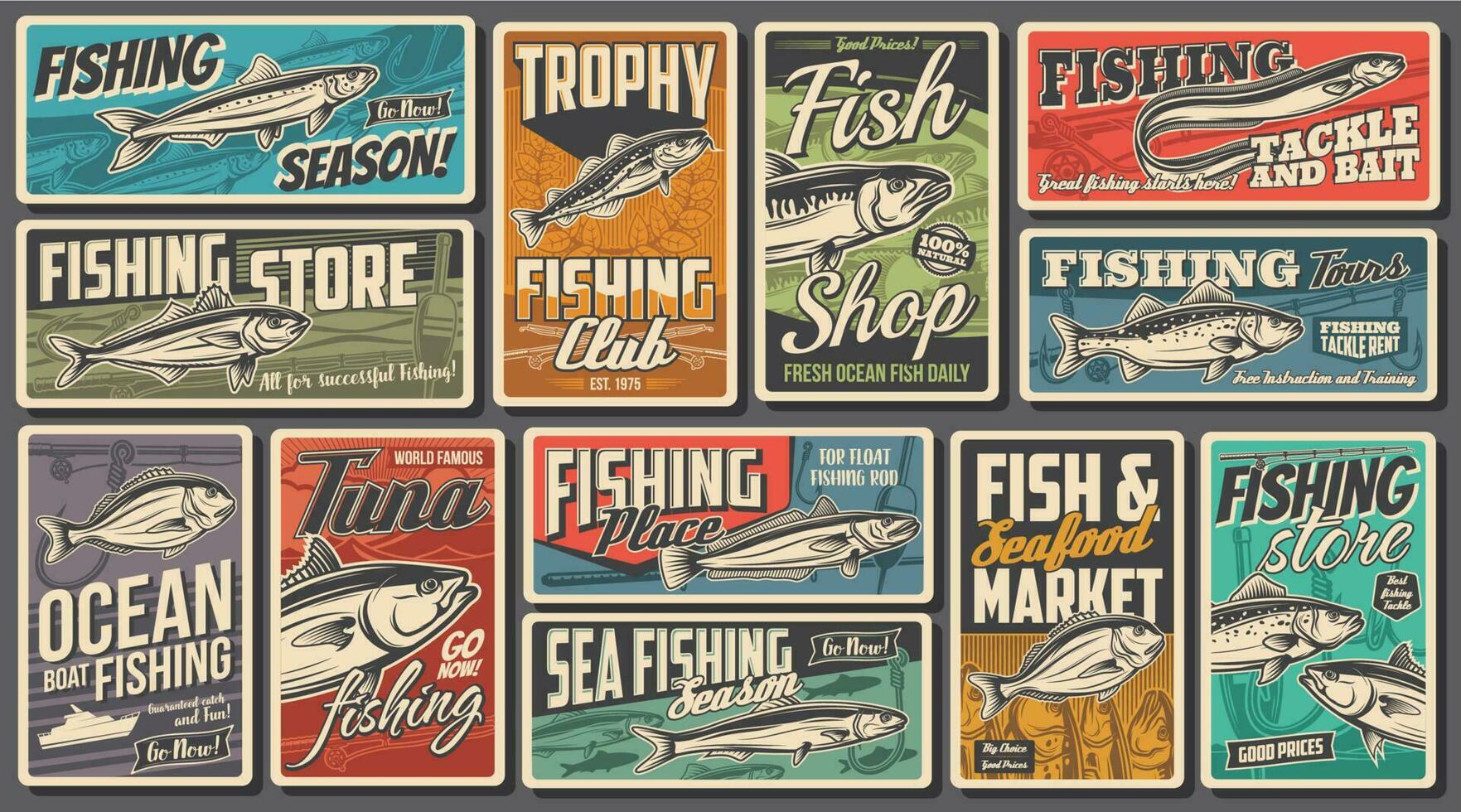The image depicts a collection of 12 brightly colored signs, all themed around fishing, mounted on a gray board. Each sign differs in color and design, but collectively they create a detailed narrative celebrating various aspects of fishing. 

In the upper left corner, one sign features a blue background with a white and blue fish and the words "Fishing Season." Below it is a similarly colored sign that reads "Fishing Store" with green lines. Adjacent is a taller, vertical orange sign proclaiming "Trophy Fishing Club" established in 1975. Next, a sign with a blue and green background offers "Good Prices" at a "Fish Shop" with "100% Natural" and "Fresh Ocean Fish Daily." 

On the upper right, another sign, colored red with an eel-like fish, states "Great Fishing Starts Here" along with "Tackle and Bait." Below, a blue sign reads "Fishing Tours," "Fishing Tackle Rent," and offers "Free Instruction and Training." To the far left bottom corner is a purple sign promoting "Ocean Boat Fishing" with a "Guaranteed Catch and Fun."

In the middle, another sign flashes "World-Famous Tuna" with the imperative "Go Now Fishing" on a red background. To its right, a sign in blue highlights a "Fishing Place for Float Fishing Rod." Underneath, on a blue and green gradient background, are the words "Sea Fishing Season" and "Go Now." Finally, a blue sign with white and yellow accents proclaims a "Fish and Seafood Market" with "Big Choice" and "Good Prices."

Each sign features different fish images, aligning with the fishing theme, and collectively, they create a visually engaging homage to the world of fishing.